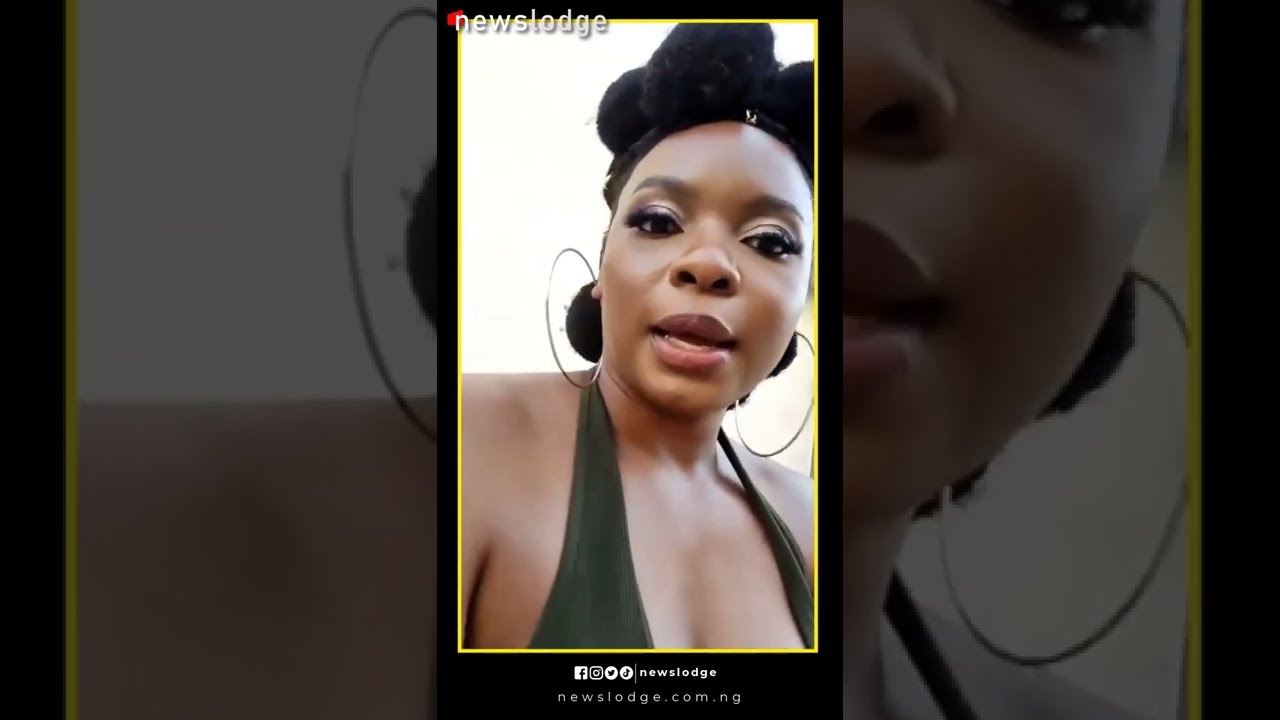In this detailed photograph featured on News Lodge (newslodge.com.ng), an African American woman is shown posing confidently. She has striking black hair styled in multiple buns, complemented by a headband that resembles a bow. Her makeup is meticulously applied, highlighting her thick eyelashes and full lips. The woman sports large hoop earrings and is dressed in a dark brown halter top or tank dress that suggests a comfort-focused style. She appears to be speaking to the camera, exuding a sense of ease.

The image is set against a white wall and is part of a triptych collage, with the main picture flanked by sections of the same image on the left and right. These sections focus on her hoop earrings and parts of her face, creating a framing effect. Above her image, the title "News Lodge" is prominently displayed in white text. Below her photo, links to Facebook, Twitter, Instagram, and TikTok are visible, further suggesting an online presence connected to this platform. The entire presentation infers that the "NG" in the website URL likely stands for Nigeria.